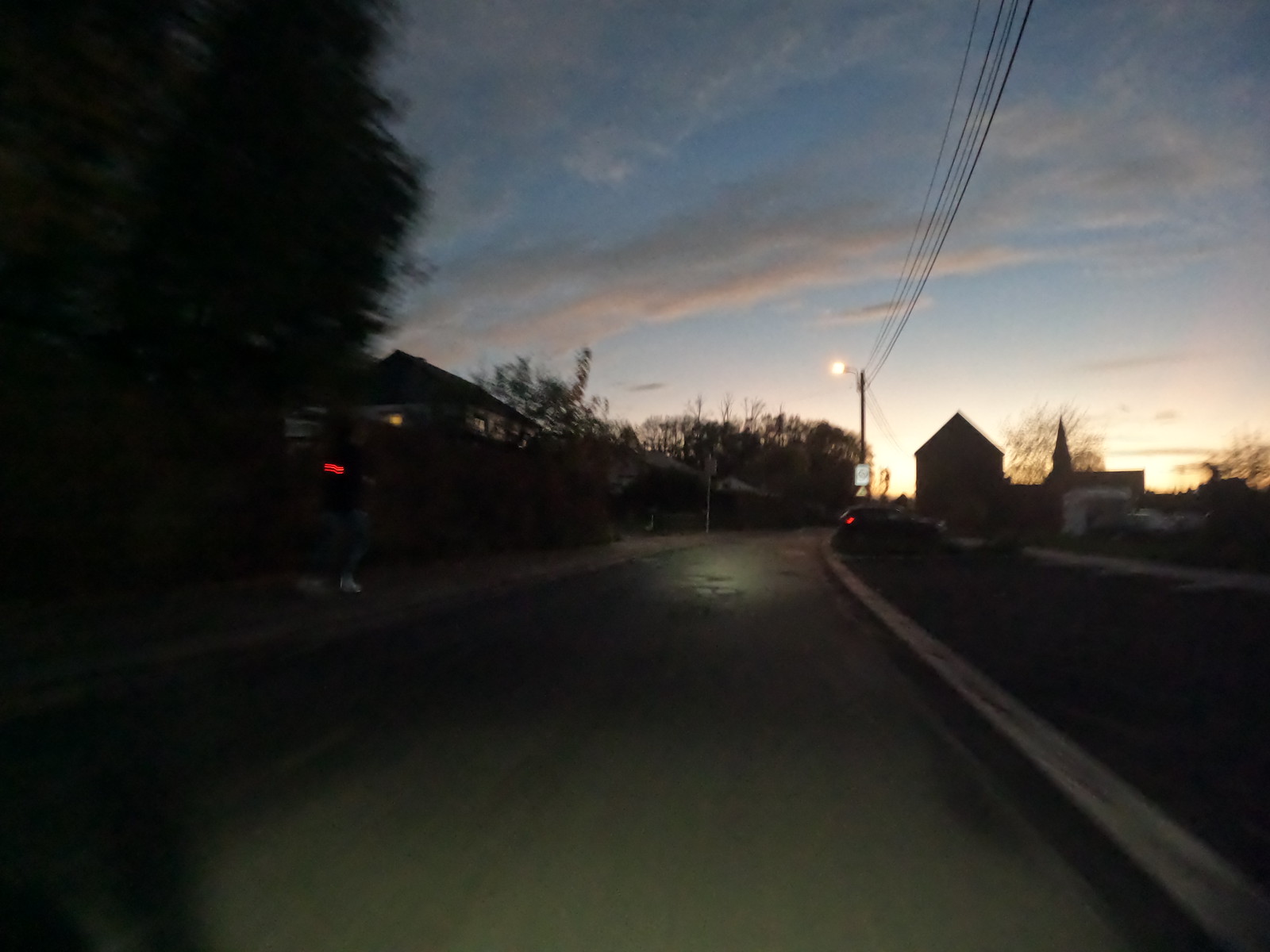The photograph captures a road scene illuminated by the dim light of either a setting or rising sun, casting an orangish glow on the horizon while the rest of the sky transitions to dark blue with scattered clouds. The road curves gently, marked by a double white line, and a single car, identifiable by its red taillight, appears to be traveling away in the distance. Silhouetted outlines of houses and trees flank both sides of the road, with a prominent tree slightly out of focus in the immediate left foreground. A streetlight, initially mistaken for the sun, is situated on a pole extending upward with electrical wires running parallel to the road. On the right side, a tree lawn, sidewalk, and snippets of a steeple suggestive of a church, alongside a home, add to the tranquil setting. Amidst these elements, a few street signs punctuate the scene, contributing to the typical yet serene dusk or dawn ambiance.